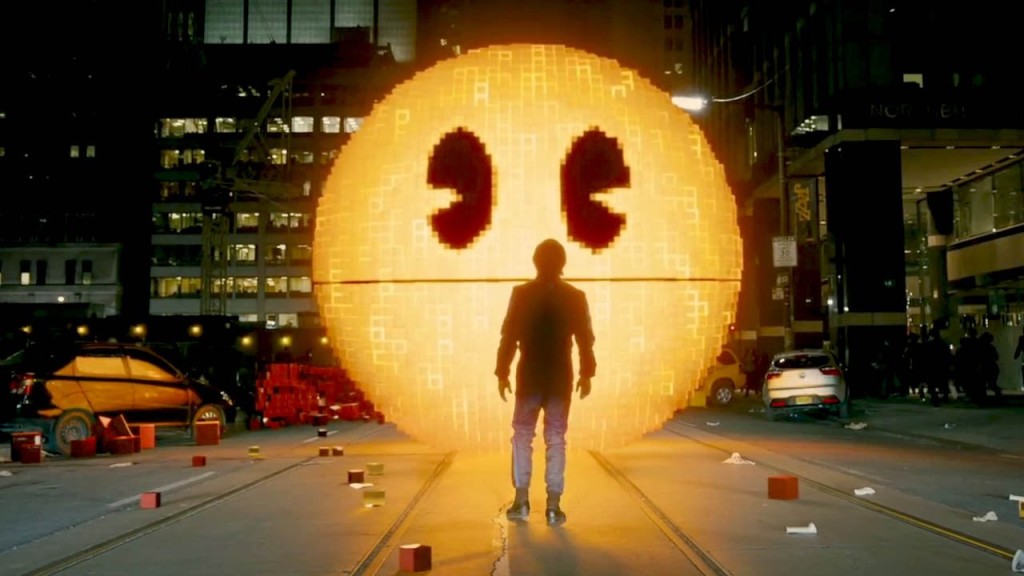The image captures a lone man standing in the middle of a rundown street in a dilapidated city. His back is to the viewer, and he is dressed entirely in dark clothing, including dark shoes, dark pants, and a dark top. The ground around him is littered with trash and scattered red bricks, alongside other white items and small red boxes. Dual cars are parked carelessly on either side of him—a black car to the left and a silver car to the right. The scene is set against a backdrop of tall skyscrapers, their numerous windows glowing with light. Centered in front of the man is a large, glowing spherical object, pixelated and yellow, resembling an orange Pac-Man or a smiley face with two black eyes. This curious, luminescent sphere captivates the man's gaze amidst the urban decay.